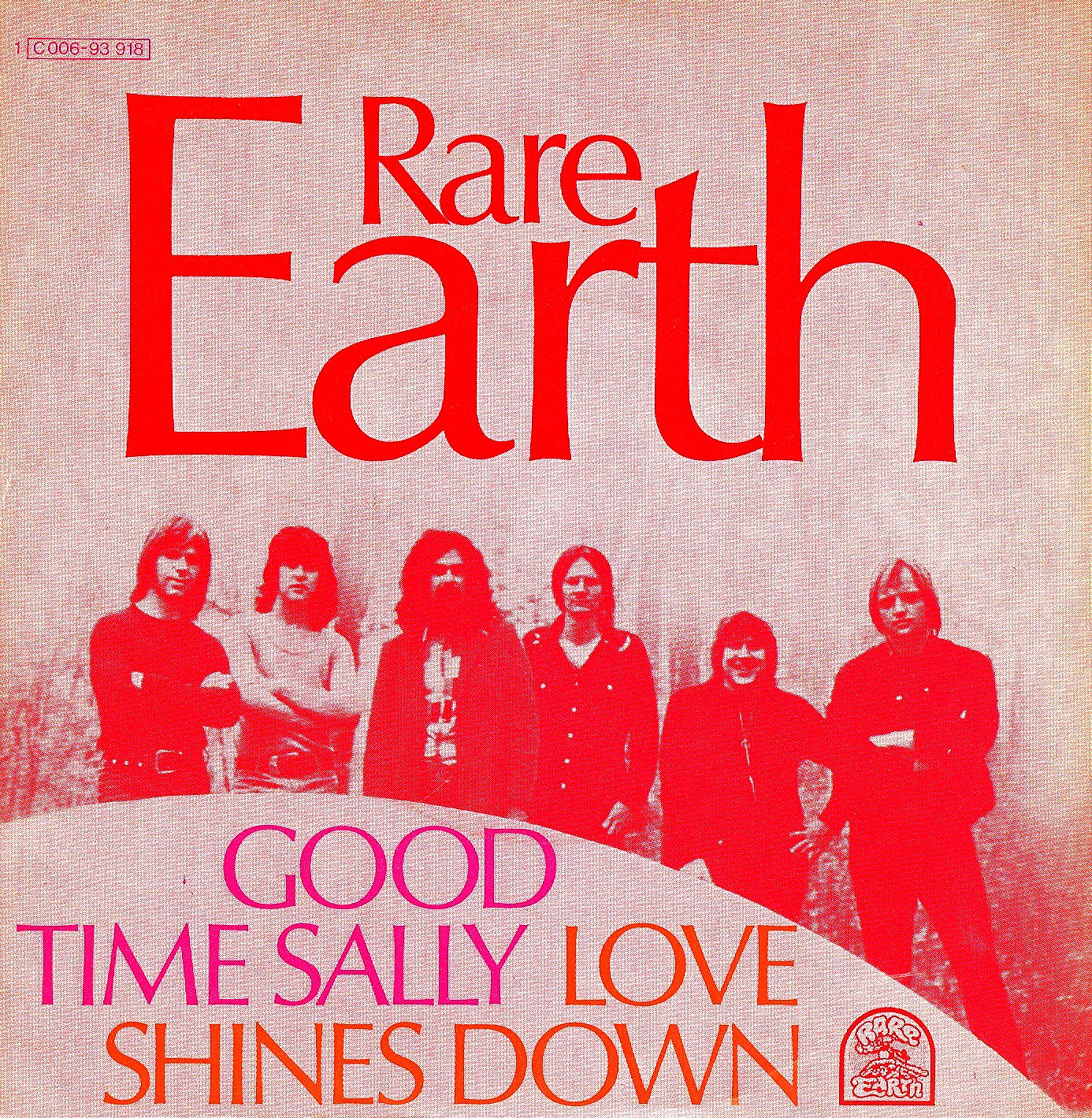The image depicts a vintage, washed-out album cover with a predominantly red, pink, orange, and white color scheme. At the top of the cover, in bold red letters, is the band's name "RARE EARTH," with "RARE" appearing above "EARTH," the latter in significantly larger font. Below this, the titles of two singles, "Good Time Sally" in pink writing and "Love Shines Down" in orange, are prominently displayed. 

Centrally positioned on the cover are six indistinct, vintage 70s band members, rendered in a grainy black-and-red monochrome style, giving them a blotched, almost eerie appearance. In the bottom right corner, a small emblem shaped like an upside-down "U" contains another "RARE EARTH" inscription, this time with red-outlined letters filled in white. This emblem features a somewhat unclear image, possibly of the earth or a train, adding to the cover's mysterious and nostalgic quality.